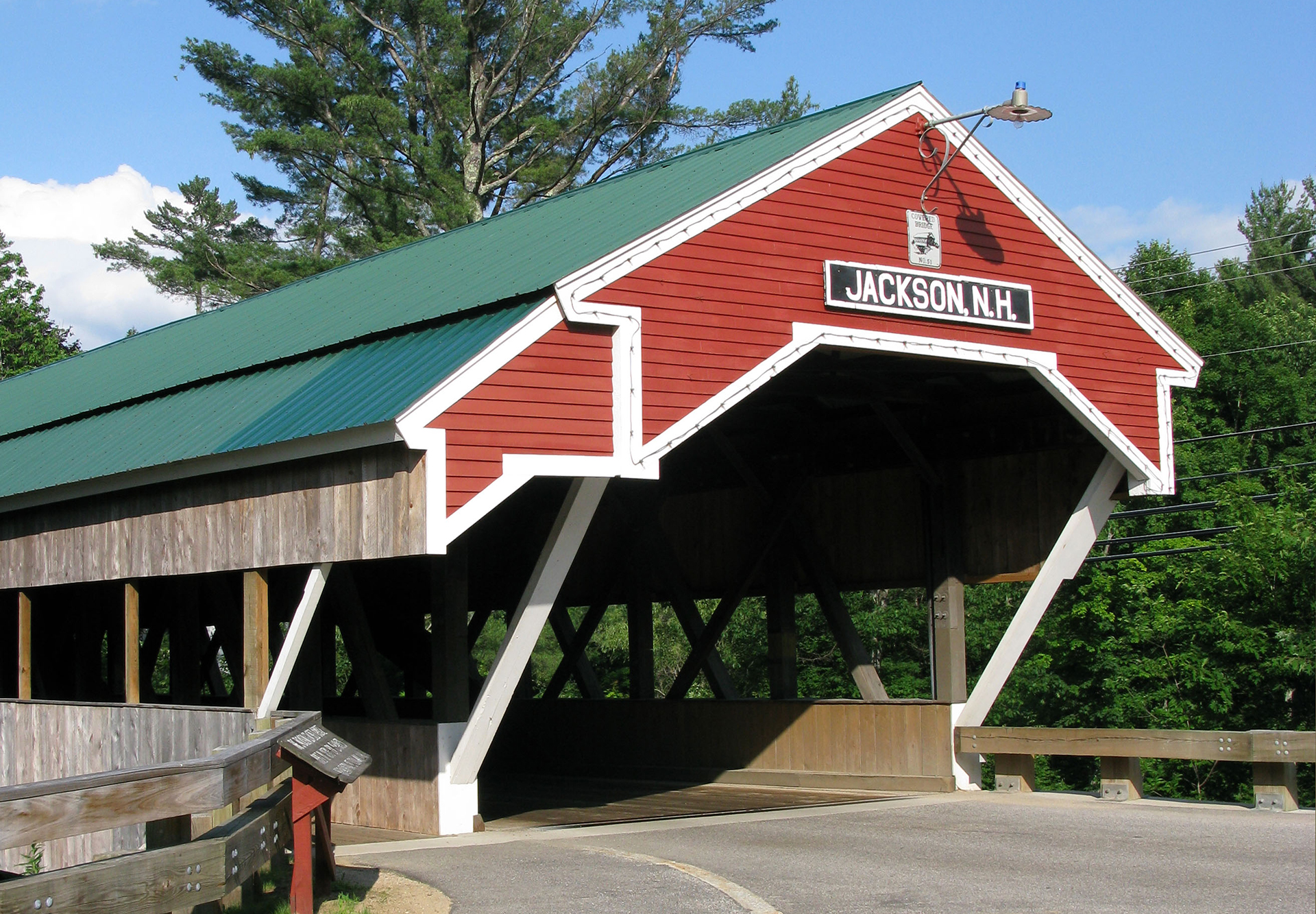The image showcases a charming old-style wooden covered bridge in Jackson, New Hampshire, identifiable by a black sign with white lettering reading "Jackson, NH" prominently displayed over its entrance. The bridge, reminiscent of a farmhouse, features a triangular peak and is adorned with a green roof composed of steeply inclined green planks. The facade facing the viewer displays a partial red section outlined in white and is supported by thick wooden beams and white support structures. Above the sign, a single bulb lamp, attached by metal bars, illuminates the sign. Although the roadway approaching the bridge is asphalt, the interior of the bridge transitions into wooden planking. The backdrop reveals a lush landscape of green trees, some of which rise above the roof of the bridge, contributing to the picturesque scene captured in daytime.